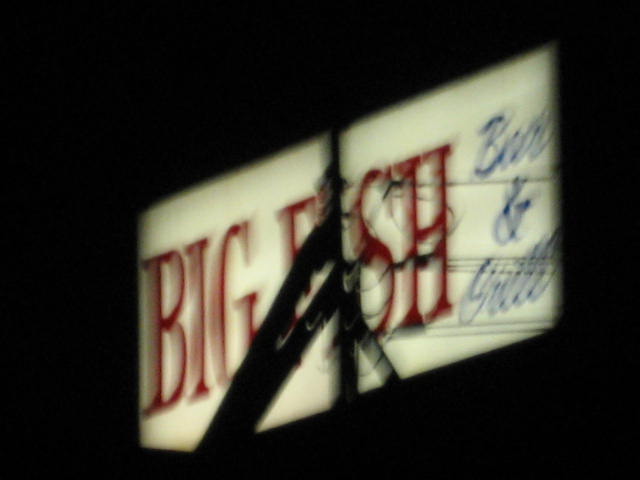The photograph, taken at night against a pitch-black background, captures a rectangular illuminated sign. The sign, glowing white, features large, capitalized red letters spelling out "BIG FISH" prominently in the center. To the right, in smaller, blue cursive text, it reads "bar & grill." The sign is slightly obscured by the silhouettes of power lines, which include insulators and cross beams that intersect in front of the sign. These power lines create a noticeable visual disruption, particularly over the letters S and H in "FISH." Despite the slight out-of-focus effect, the details on the sign remain clear and readable.